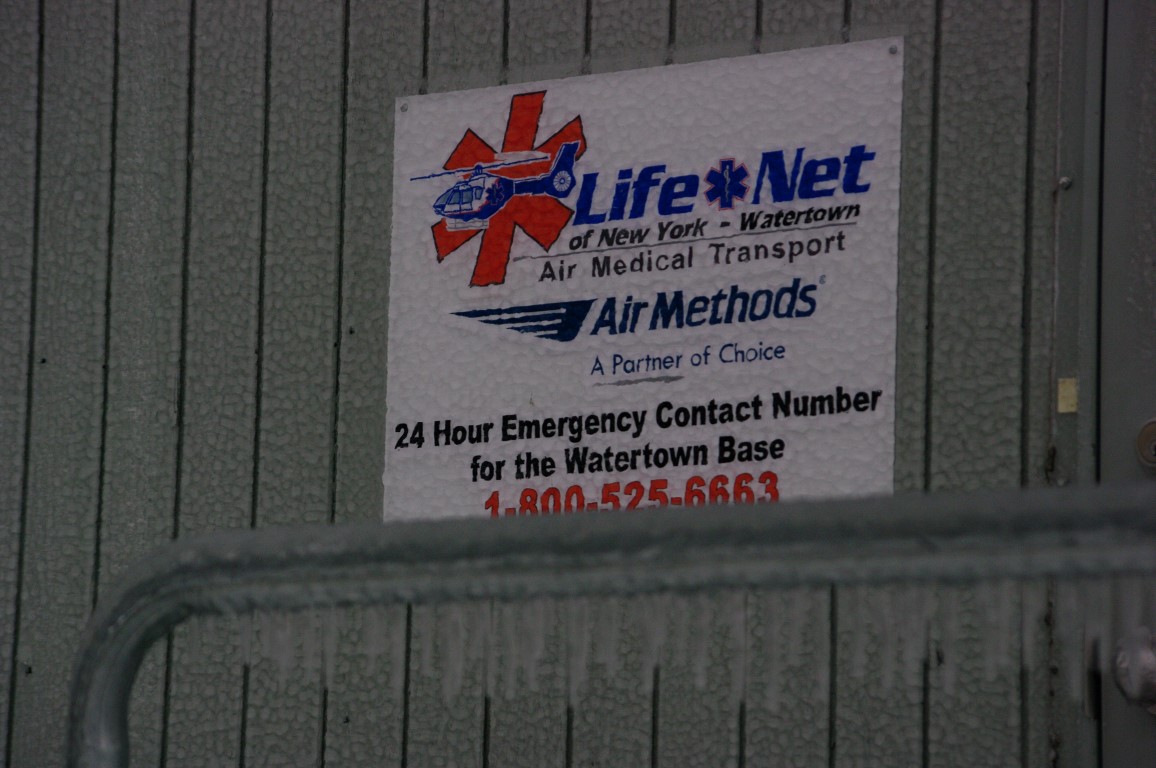The photograph captures the side of a wooden building with vertical siding that has a greenish hue. A white sign with red, blue, and black text is prominently displayed, screwed into the wood. The sign, accented by a red asterisk behind a blue helicopter logo, reads: "LifeNet of New York, Watertown, Air Medical Transport, Air Methods, a partner of choice." Further detailed text at the bottom of the sign includes a 24-hour emergency contact number for the Watertown base, listed as 1-800-525-6663. In the foreground, a curved silver handrail adorned with frozen ice and icicles, dripping like popsicles, suggests the photograph was taken during winter.